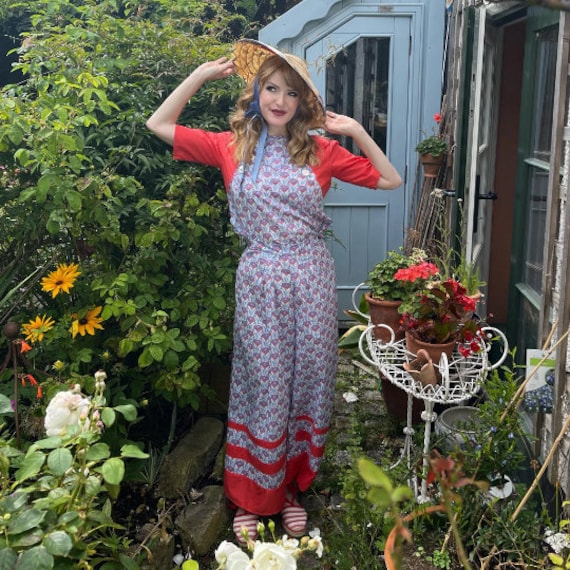In the center of the photograph stands an attractive young blonde woman, appearing to be in her late 20s or 30s, and radiating happiness with a smile or smirk as she looks off to the left. She is adorned in a long dress featuring a floral pattern with purple flowers interspersed with shades of blue and white. The dress has striking red borders at the bottom and is complemented by a red shirt that peeks out underneath, covering her upper arms and shoulders. Her footwear is a pair of white espadrille shoes lined with dark red stripes. Adding to her summery look, she wears a straw sun hat, jauntily angled and secured with a blue bow under her chin, with her fingertips resting lightly on its brim.

The woman is set against a vibrant garden backdrop, possibly adjacent to her home or a greenhouse, characterized by tall green plants and vivid sunflowers. To her right, a white stand displays various potted flowers, adding to the botanical ambiance. Behind her, a light blue door—part of a larger structure that extends off the image and includes a visible window—provides a charming and serene setting that frames her joyfully.